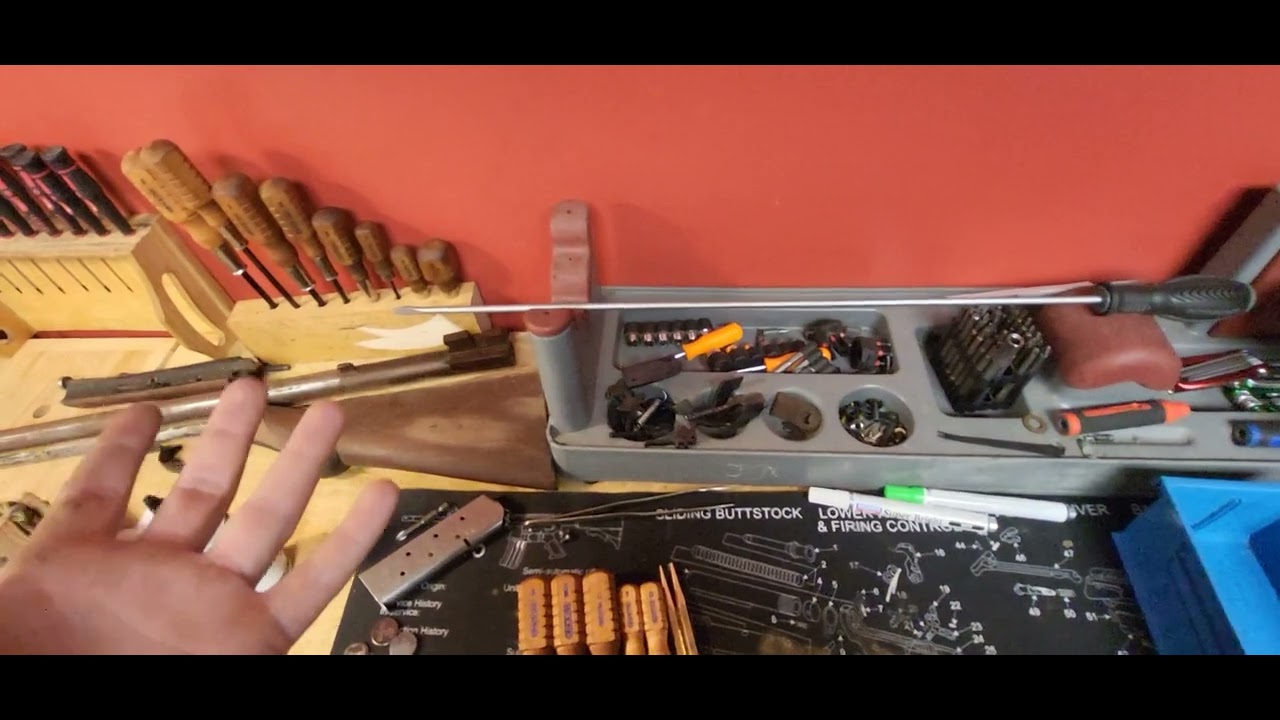This photograph captures a cluttered and detailed workspace centered around a natural wood workbench set against an orange-red rear wall. Dominating the scene is a myriad of hand tools, including precision screwdrivers and awls, some mounted vertically in wooden holders on the left. In front of these, small drill bits and screws can be seen scattered within a silver tray. A large silver chisel with a black handle lays prominently among the tools. A symmetric blue box frame is positioned on the lower right, and a black mat with the partially visible words "Sliding Buttstock, Lower and Firing Control" written in white letters spans the center. Overlaying the text are various pens, adding to the disordered feel. In the lower left corner, a person's left hand rests palm-up, gesturing towards the tools, possibly showcasing the collection. A partially visible gun buttstock peeks out in the foreground, suggesting that the space is used for the building or repairing of weapons.